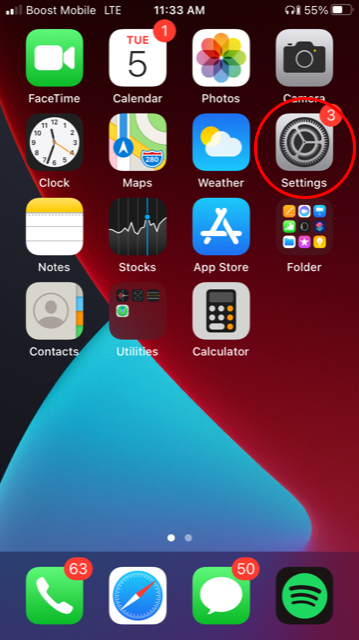This image is a high-resolution screenshot taken from an iPhone, specifically showing the home screen. At the center of attention is the Settings application, clearly indicated by a gray gear icon encircled in red. This addition suggests the image’s intention is to draw focus to the Settings app. 

The background of the home screen fades between shades of red, blue, and black, creating a visually striking gradient. At the bottom dock of the screen, there are four primary apps: the green Phone icon with a notably high count of 63 notifications, the blue Safari browser represented by a compass icon, the Messaging app displaying 50 unread messages, and the Spotify app featuring its characteristic green icon.

The home screen displays the first of two pages, populated with a range of default and third-party apps. The top row includes FaceTime and Calendar, the latter bearing a single notification badge. Further down, we see familiar utilities such as Photos, Camera, Clock, Maps, Weather, and the central Settings app, which also has three pending notifications. Below these are the Notes, Stocks, App Store, and Contacts apps. Additionally, there are two self-made folders: one houses miscellaneous apps, while another contains utility apps. The Calculator app rounds out the lower portion of the screen.

All elements combined offer a comprehensive representation of the user’s primary apps and notifications, with a distinct emphasis on the Settings icon.